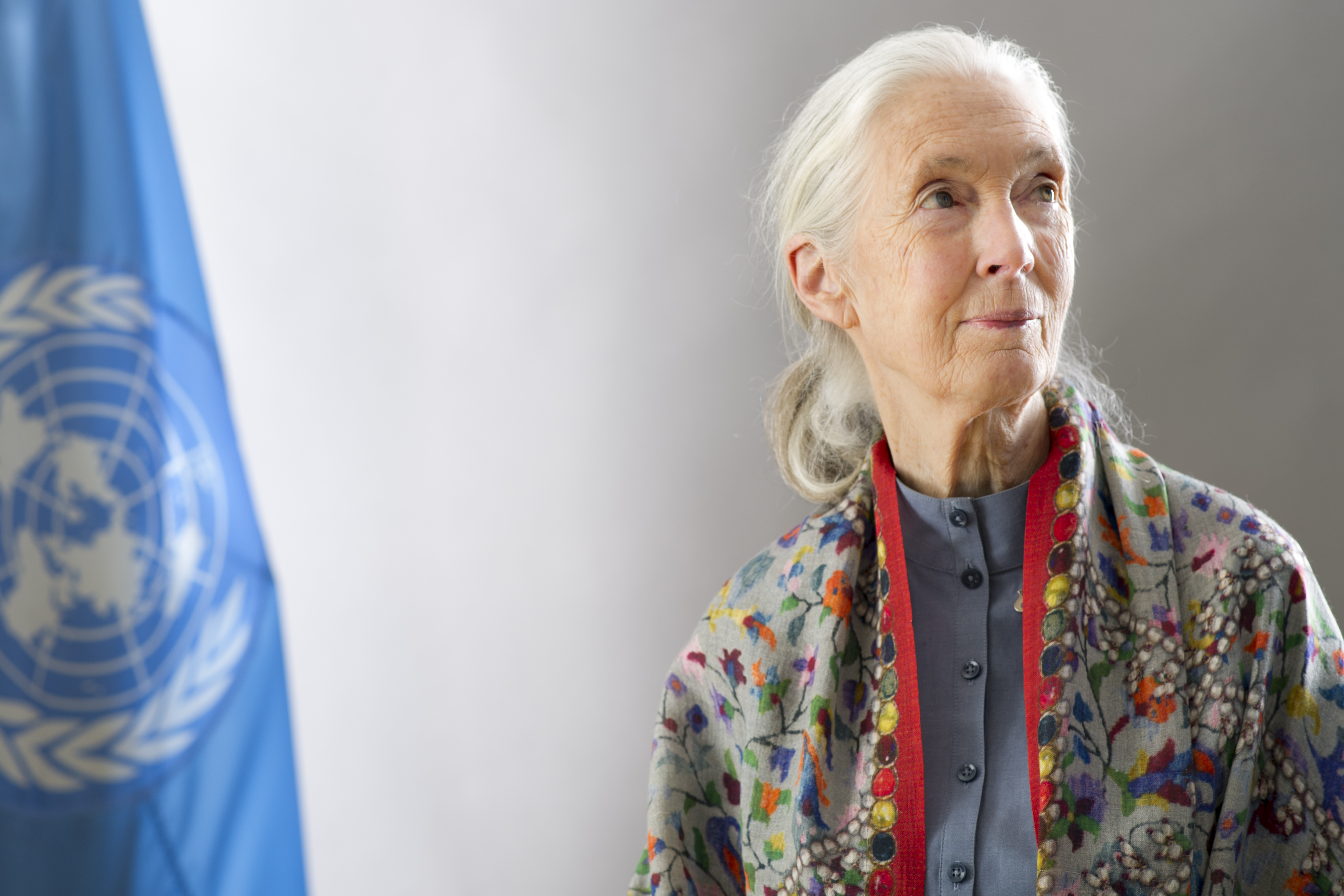The image depicts renowned primatologist Jane Goodall standing slightly to the right side, gazing upward toward the top right of the frame. Jane's silver-gray hair is pulled back into a ponytail, behind her head. Her face is marked with the wisdom of wrinkles, and her light-colored eyes convey a thoughtful expression. She is clad in a bluish-gray, high-collared button-up shirt, resembling a mock turtleneck, peeking out beneath a highly decorative cardigan adorned with intricate patterns. The cardigan features floral designs, branches, birds, and red trim, with additional colorful dots and abstract bead-like illustrations enhancing its vibrant aesthetic. In the background to the left, though slightly out of focus, is the blue and white flag of the United Nations, showcasing a central globe encircled by olive branches, adding a context of international recognition and significance to the photograph. The backdrop is a plain gray, which contrasts elegantly with her striking and detailed attire.